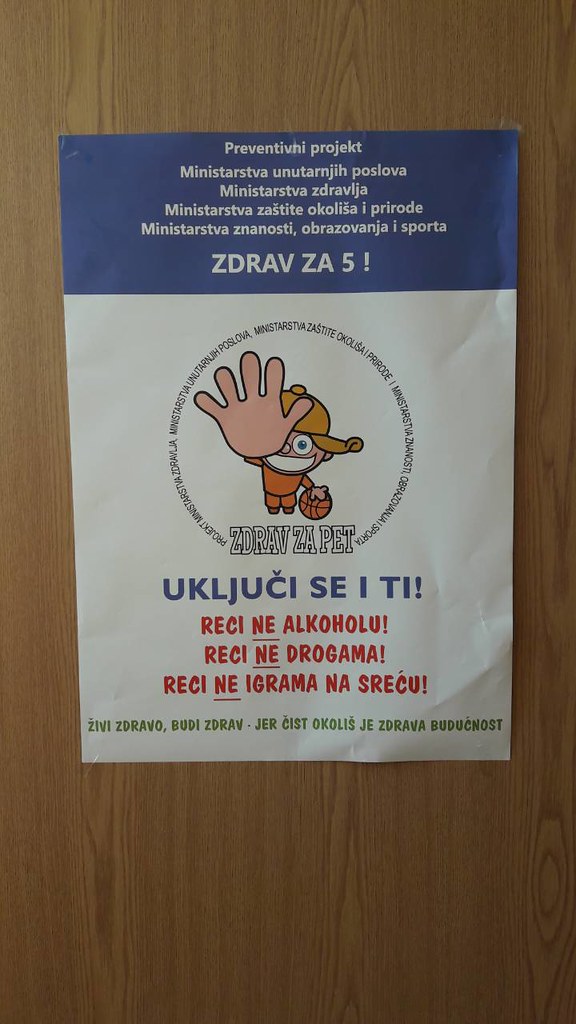The image depicts a wrinkled flyer taped to a light brown, wood-patterned door. At the top of the flyer, a blue section bears white text that reads "Preventivny Project Ministarstva Unitarnej Poslova," indicating a preventive project by a ministry. Below this, additional white text appears on a white background, accompanied by a cartoon drawing of a smiling boy at the center of a circle. The boy, who has a large grin and big eyes, is wearing a tan and orange outfit. He has a cap on, one hand on a basketball, and his other hand extended outward, palm facing the viewer. The circle encircling the boy is composed of small words. Beneath the boy, the text "Z D R A V Z A P E T" is prominently displayed, followed by a line of blue letters and three lines of red letters. At the very bottom of the flyer, there is another line of text in a beige color that spans the entire width of the paper. All the text is in a foreign language.